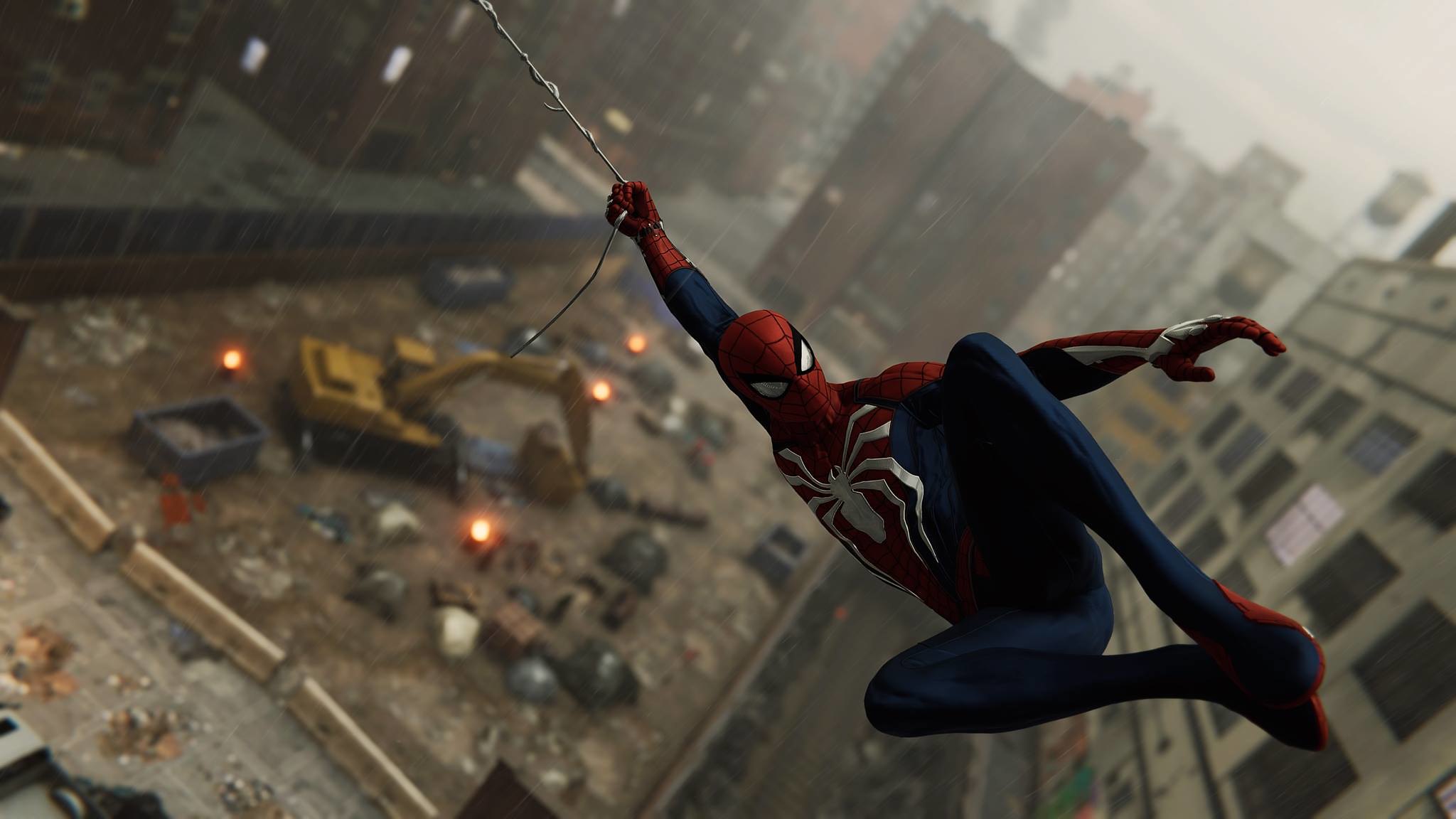In this animated or video game scene, Spider-Man is prominently featured in the foreground, dynamically suspended by his right hand from a web descending from the top of the image. His iconic red and blue suit, adorned with a silver spider emblem on his chest, stands out. Spider-Man's left arm extends outward, while his legs are pulled up to his body, with his feet together and knees spread apart, creating a sense of motion as he swings. His mask, with its pronounced silver eye lenses, faces forward, directly engaging the viewer.

Below him to the left, a fenced-off construction site dominates the middle ground. This area is filled with dirt and equipped with various items: a large yellow excavator, orange lights, dumpsters, and large containers. Yellowish concrete barriers mark the boundary between the lot and a nearby street. In the background, tall buildings blur into a grey and gloomy sky, contributing to a rainy, slick atmosphere devoid of cars. This urban scene intensifies the action-packed yet somber mood of the image.